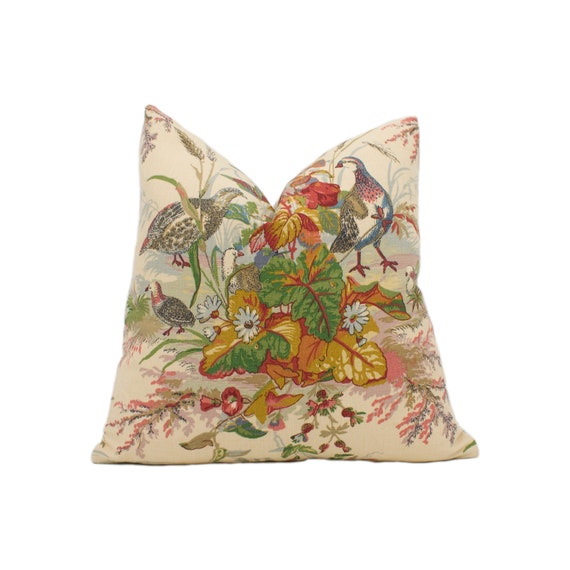The image depicts a beige throw pillow, slightly crumpled and set against a white background, with an intricate and vibrant oriental print. The pillow features an embroidered pattern with a variety of elements: several types of colorful birds, including what appears to be a white duck, a quail, and a larger bird with blue, navy, and pink hues around its neck. Alongside the birds are green ferns, leafy plants with veined leaves that exhibit shades of green and yellow, and small white daisy-like flowers. Additionally, there are delicate pink and red blossom branches scattered throughout the design, contributing to the rich, detailed tapestry of flora and fauna on the pillow.